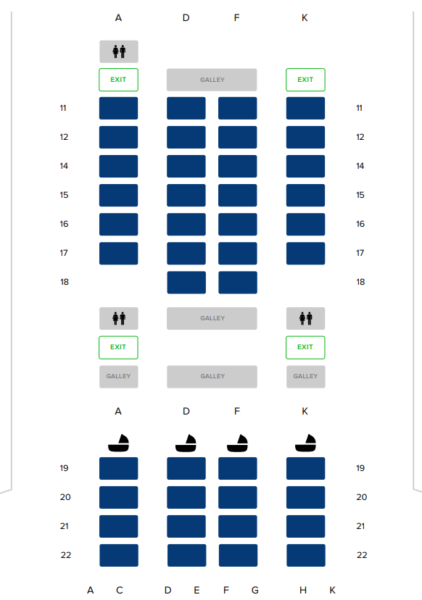This image is a screenshot of an application or website intended for selecting seats or rooms. The layout closely resembles that of a cruise ship but could potentially apply to other types of transportation or venues like an airline, concert hall, or ferry. However, several elements suggest a maritime context.

The interface features a clean, white background with light gray lines running vertically on the left and right sides. The screenshot is cropped, making it unclear whether it was taken from a browser or a mobile device, as it lacks visible UI elements typical of either.

At the top of the layout, the content is organized in a grid with four columns labeled A, D, F, and K. Column A starts with a gray rectangle displaying the male and female bathroom symbols, followed by a green outlined rectangle with a white interior and green text reading "Exit". Below these, there are six uniformly sized blue rectangles. After a small gap, another bathroom icon appears, followed by another green exit rectangle. Further down, there is a gray rectangle labeled "Galley" in light letters. Continuing, there's another set of four blue rectangles labeled under the letter 'A', and finally, a boat icon, reinforcing the notion that this layout is related to a maritime vessel.

Adjacent to Column A in Column B, the layout includes sequential labeling of rows numbered 11, 12, 14, 15, 16, 17, 18, followed by a space, and then continuing with rows 19, 20, 21, and 22.

Columns D, F, and K mirror the arrangement in Column A but do not include bathroom icons. The repetitions and specific layout nuances strongly hint that this configuration is part of a larger seating or room arrangement suitable for a cruise ship's deck plan.